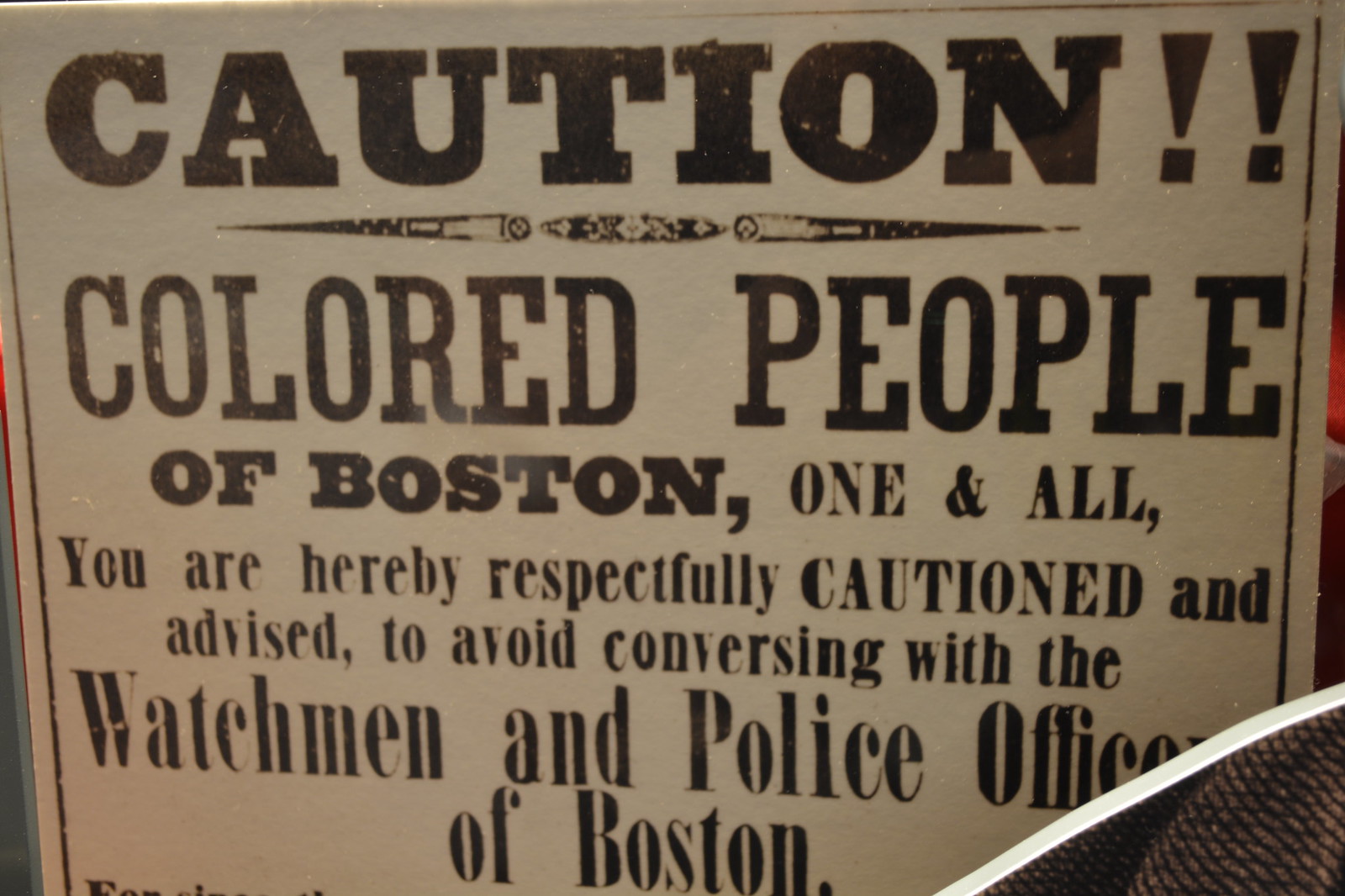This is a close-up photograph of a vintage sign with a slightly dull, whitish background and bold black text. At the top, it reads "CAUTION!!" in all-uppercase letters. Below that, there is a decorative element consisting of an oval flanked by small triangles with circular bases pointing left and right. Underneath the decoration, the sign reads "COLORED PEOPLE OF BOSTON" in bold text, with "one and all" following in smaller, less bold letters. The main body of the text states, "You are hereby respectfully cautioned"—with "cautioned" in bold, uppercase letters—and continues, "and advised to avoid conversing with the watchmen and police officers of Boston." The word "officers" is partially cut off at the bottom right by a white line extending diagonally. Additionally, the letter "N" in "Boston" is also slightly cut off. Below this text, there is a pattern that resembles snake skin.